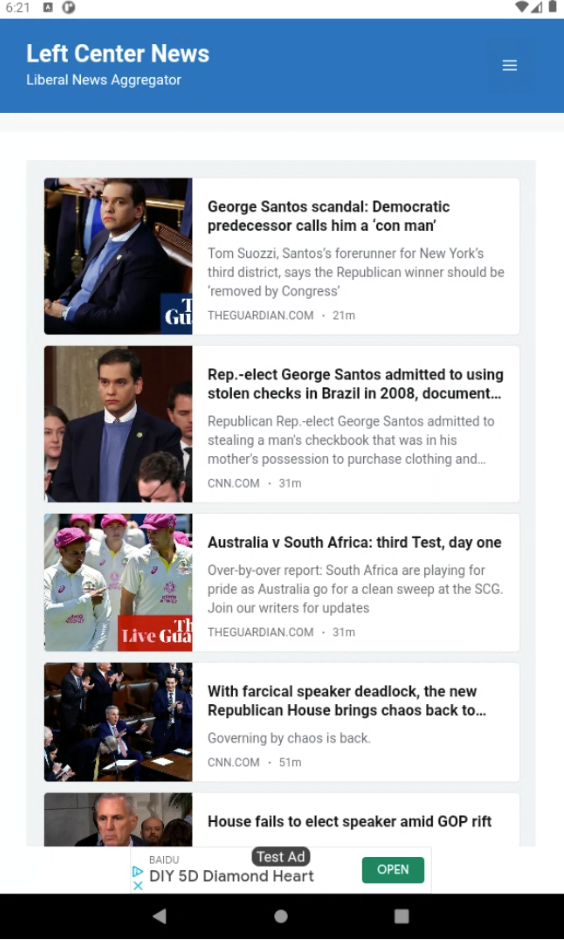The image presents a detailed view of a news website named "Left Center News," clearly catering to Democratic news as indicated by its tagline, "Liberal News Aggregator," situated beneath its name in white text on a blue background in the top left corner. The top portion of the website is set against a deep blue background, giving way to a dominantly white central area that serves as the main content section.

In the center of the page, the content is organized with article images on the left and corresponding text descriptions in black on the right. In total, there are five articles displayed. For the top article, there is a photograph of a man in a suit, seemingly in a seated position. To its right, the headline reads "George Santos Scandal" with a sub-caption, "Democratic predecessor calls him a con man," focusing on an unfolding political controversy.

Beneath the articles, at the very bottom of the website, there is a solid black bar. The layout aesthetically separates different segments, ensuring clarity and visual structure. This comprehensive, visually ordered approach underscores the website's aim to present information clearly to its predominantly Democratic readership.